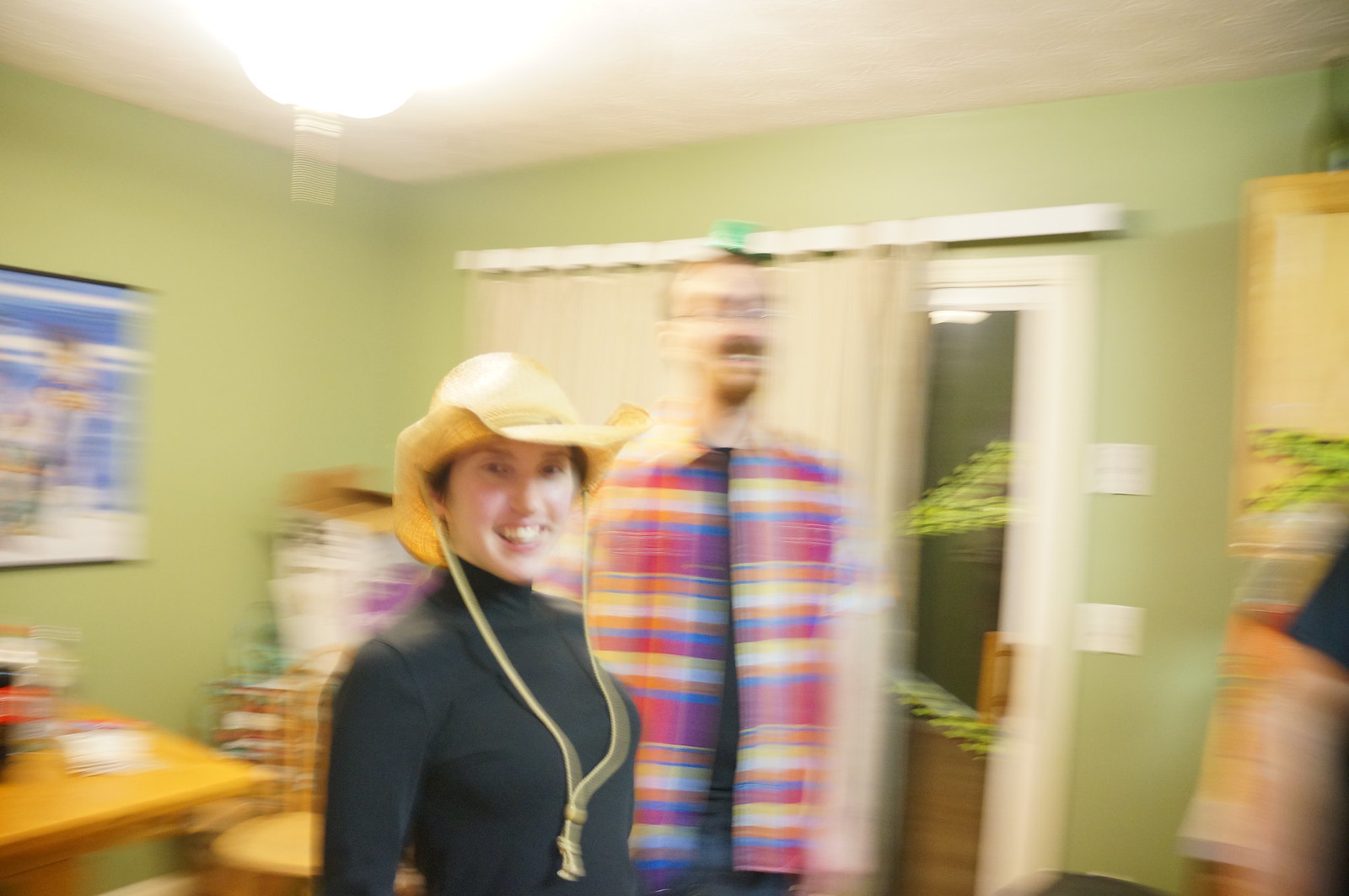In this blurry indoor photograph, likely taken with a moving camera, two individuals are captured against a lime green wall illuminated by a bright ceiling light. On the left, a woman is seen wearing a black long-sleeve shirt and a cowboy hat with matching rope ties that hang loosely across her chest. To her right stands a man, distinguished by his goatee, glasses, short hair, and a checkered red scarf draped around his neck. The overall scene is somewhat indistinct but vibrant, with the light enhancing the green hue of the background.